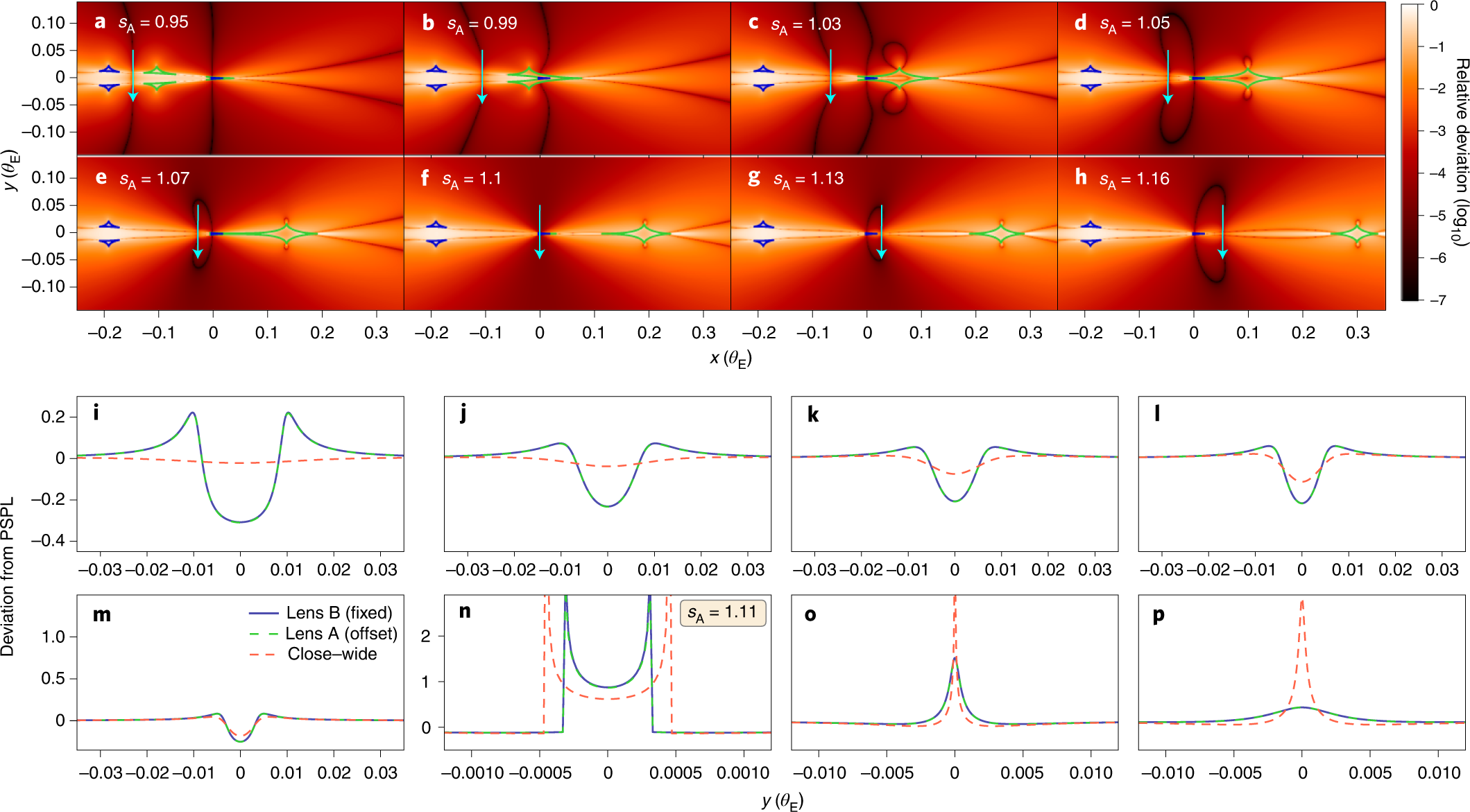The image showcases a detailed scientific visualization consisting of multiple types of charts. At the top, there are eight thermal scans in different colors including orange, brown, and black, displaying a variety of data forms. Accompanying these scans is a legend in the upper right corner, labeled "relative deviation, log 10," which transitions from white to black. Below these thermal scans, the image features several line graphs against a white background with both green and red dashed lines. The green lines are predominantly straight but exhibit various bends and tips in the middle, indicating data deviations. The overall layout suggests an analysis involving deviation from PSPL, emphasizing some sort of scientific phenomenon captured through these charts and graphs.